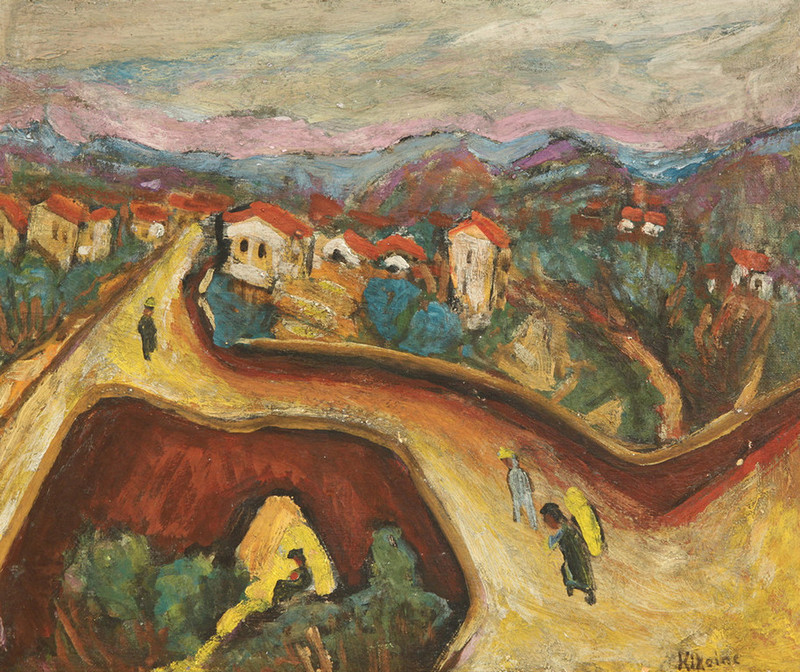This intricate painting showcases a bustling village scene with pathways winding through clusters of Spanish-style houses, characterized by beige walls and orangish-red roofs. The roads meander from the lower right corner, extending towards the horizon, which is adorned by a picturesque mountain range under a blue and pink sky. In the artwork’s foreground, a field encircled by trees, shrubs, and bushes occupies the lower left portion, lending a lush green contrast to the landscape. Along the pathway, several villagers can be seen: four people in distinct attire – one in black, another in yellow, one in white, and another in black. They navigate the curved, wavy roads that lead to various parts of the village. The scene, reminiscent of French Impressionist style with predominant browns, yellows, and blues, immerses viewers in a timeless, dynamic atmosphere.